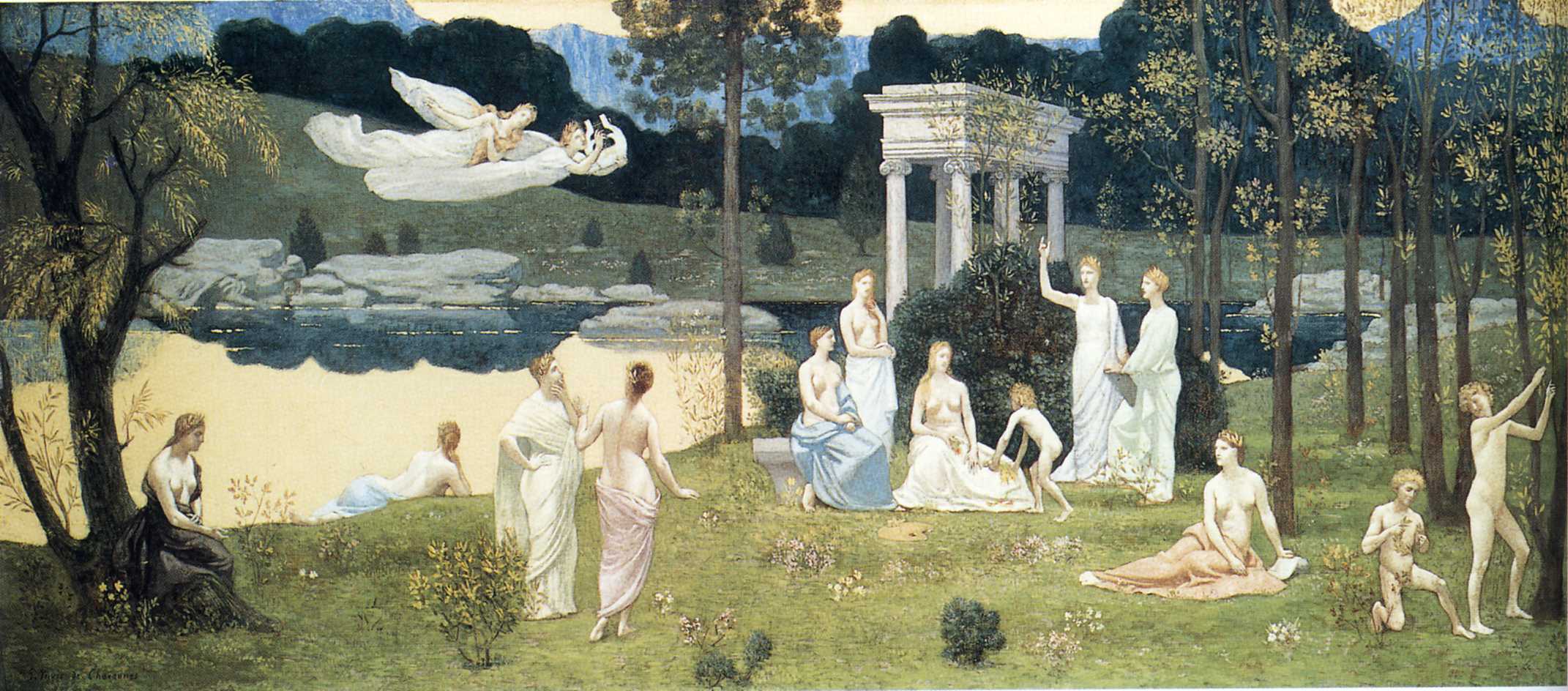The painting, which dates back at least a century or two, presents a detailed and somewhat realistic depiction of a serene lakeside scene, possibly inspired by ancient Greek times. The focal point is a group of approximately 10 to 15 individuals, predominantly women, scattered along the grassy banks of a lake or pond. Some are unclothed while others are draped in long, white gowns or togas, indicating a classical setting. 

To the left, amidst the lush greenery of trees with leaves in shades of green and yellow, angels hover above the scene, two of them playing instruments, adding a celestial ambiance to the tranquil setting. A notable architectural structure resembling a classical Greek temple with columns and a shaded area stands in the background, lending an air of antiquity to the landscape.

The foreground features rocks near the water's edge, with people positioned centrally around them, either sitting or standing on the grass. The backdrop includes a tree row and distant mountains, creating a layered and picturesque composition. The lake itself appears blue, contrasting with the verdant surroundings.

The painting's medium could be watercolor or oil-based, given its vibrant yet realistic portrayal of the landscape and figures. Overall, the artwork exudes a timeless, serene beauty that blends natural and mythological elements seamlessly.